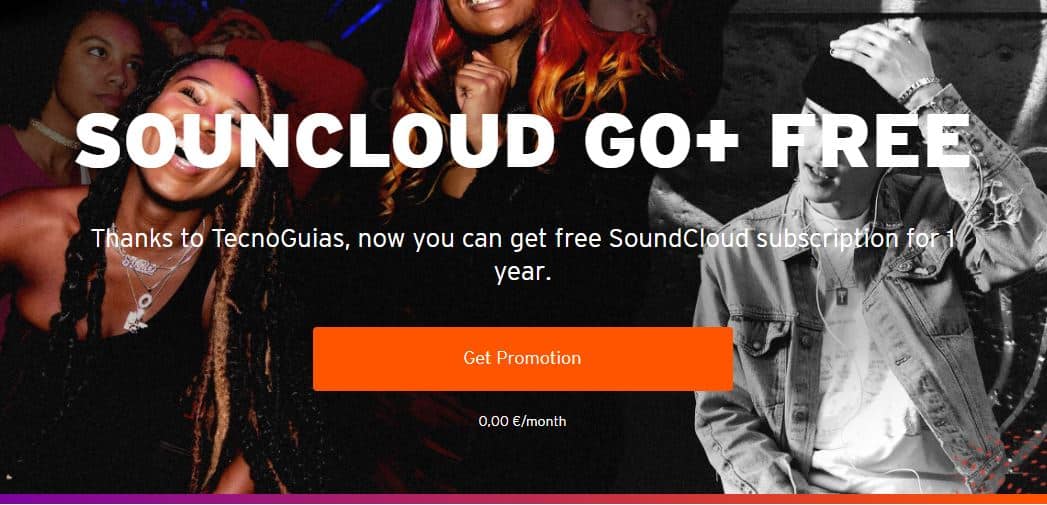The advertisement I am currently viewing for SoundCloud Go Plus Free features a vibrant and energetic scene as its background. This backdrop showcases a group of three to four women and one man, all dressed up and seemingly enjoying a night out at a lively nightclub. The atmosphere is festive and full of life, aligning perfectly with the upbeat nature of the promoted service.

Overlaying this lively image is a bold white text proclaiming "SoundCloud Go Plus Free" at the top, making the purpose of the ad immediately clear. Further enhancing the offer, another line of text states, "Thanks to Techno Gaius, now you can get a free SoundCloud subscription for one year," adding a sense of exclusivity and urgency to the promotion.

To make the deal even more enticing, there's an orange 'Get Promo' button prominently placed at the center below the text, inviting users to click and avail the offer of $0 per month for a year-long SoundCloud Go Plus subscription. The design elements are strategically positioned to draw attention to the key message and call-to-action, ensuring that potential subscribers don’t miss the opportunity to benefit from this generous promotion.